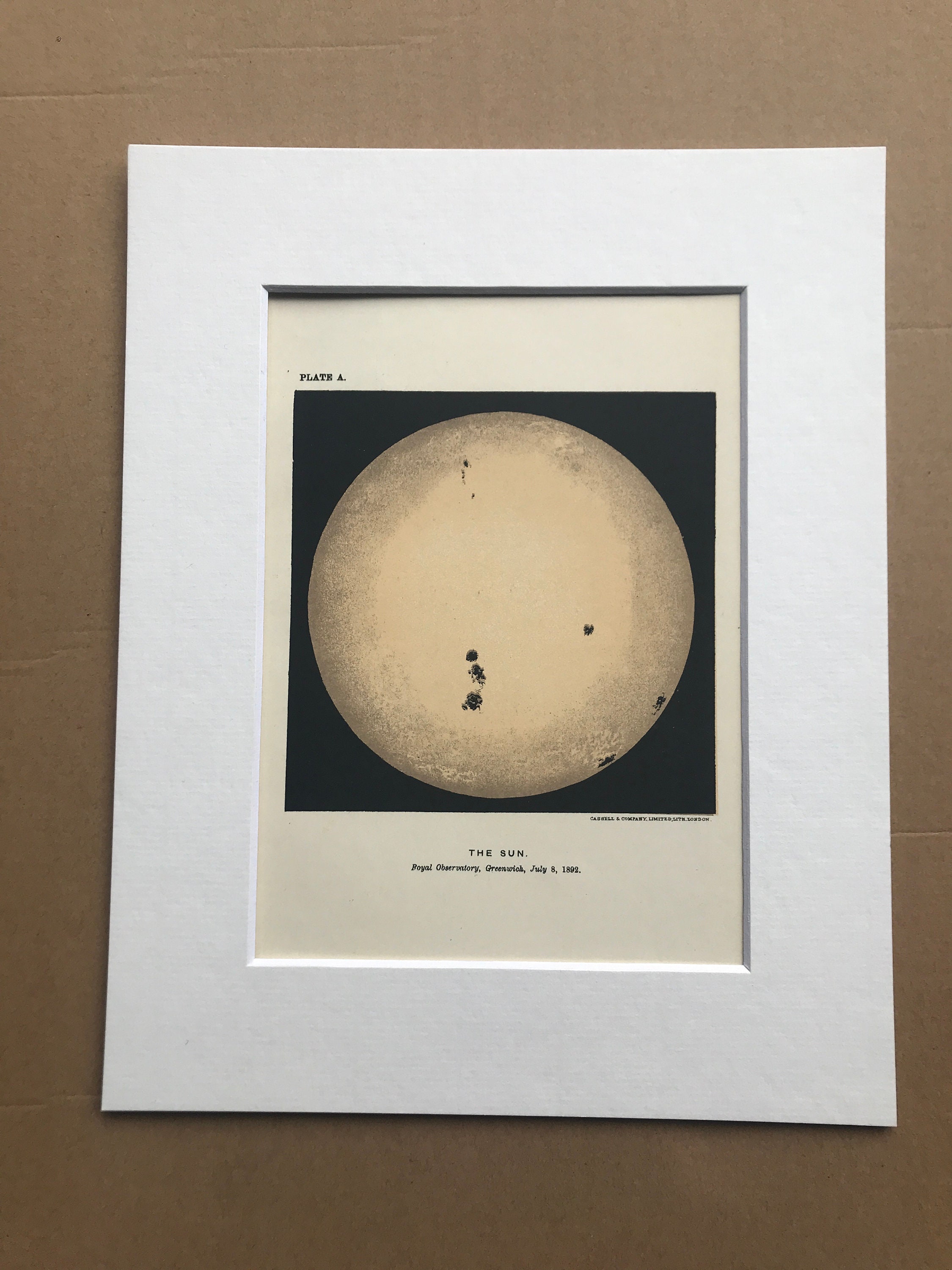This vertical rectangular image features a double-matted, framed picture labeled "The Sun." The outermost boundary is a dark brown rectangle, which frames a slightly off-center white matting. Inside that is another white mat that appears to be part of the picture's composition. The inner picture shows a black square with a circular object, predominantly white with black spots, labeled "The Sun." Additionally, the object has three distinct spots in the lower part.

The text below the image reads "The Sun" in all capital letters, followed by "Royal Observatory Greenwich July 8th, 1892" in regular text. The background surrounding the frame is dark brown. The circular object, initially mistaken for the moon, is confirmed as the Sun upon closer inspection. The black spots on it are identified as sunspots, adding to the celestial detail of the framed print.